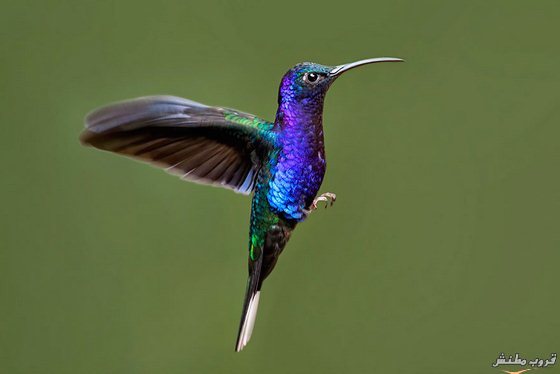In the center of this photograph, a hummingbird is captured mid-flight against a completely green, likely blurred background. The bird, appearing to be in the process of landing, has both wings extended behind its back and both feet positioned downward in a c-shape. Its feathering is predominantly blue, with patches that transition into a vivid purple, particularly around its neck. Its long, thin black beak and distinctive tail feathers which transition from greenish to black, ending in white tips, are clearly visible. The scene seems to be set outdoors, possibly during the day. In the bottom right corner of the image, there is small, hard-to-read white text that appears to be in Arabic, adding an international element to the photograph.